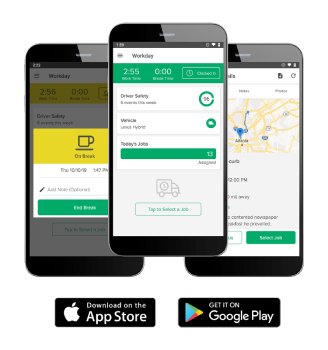The image features a promotional advertisement showcasing three iPhones arranged artfully. Two iPhones lie flat in the background, partially covered by a third iPhone in the foreground, which sits atop them and covers their right and left-hand sides. Below the iPhones, there are promotional buttons for app downloads: the "Download on the App Store" button with the Apple logo and the "Get it on Google Play" button with the Google Play logo.

The iPhone on the left displays an app called "Workday." The screen shows a notification bar with a yellow banner and an icon of a coffee cup that reads "On Break." Additionally, numbers "255" and "0" are seen, suggesting some form of status count, although the precise context is unclear.

The iPhone in the center has a gray icon of a panel truck, accompanied by a green button below it, which is illegible.

The iPhone on the right features a map at the top of its screen, with some unreadable text beneath it. A white and green button is visible at the bottom of this screen but is too blurred to decipher. The overall scene implies a promotional focus on productivity and logistics apps, highlighted by the accompanying download buttons for the App Store and Google Play.